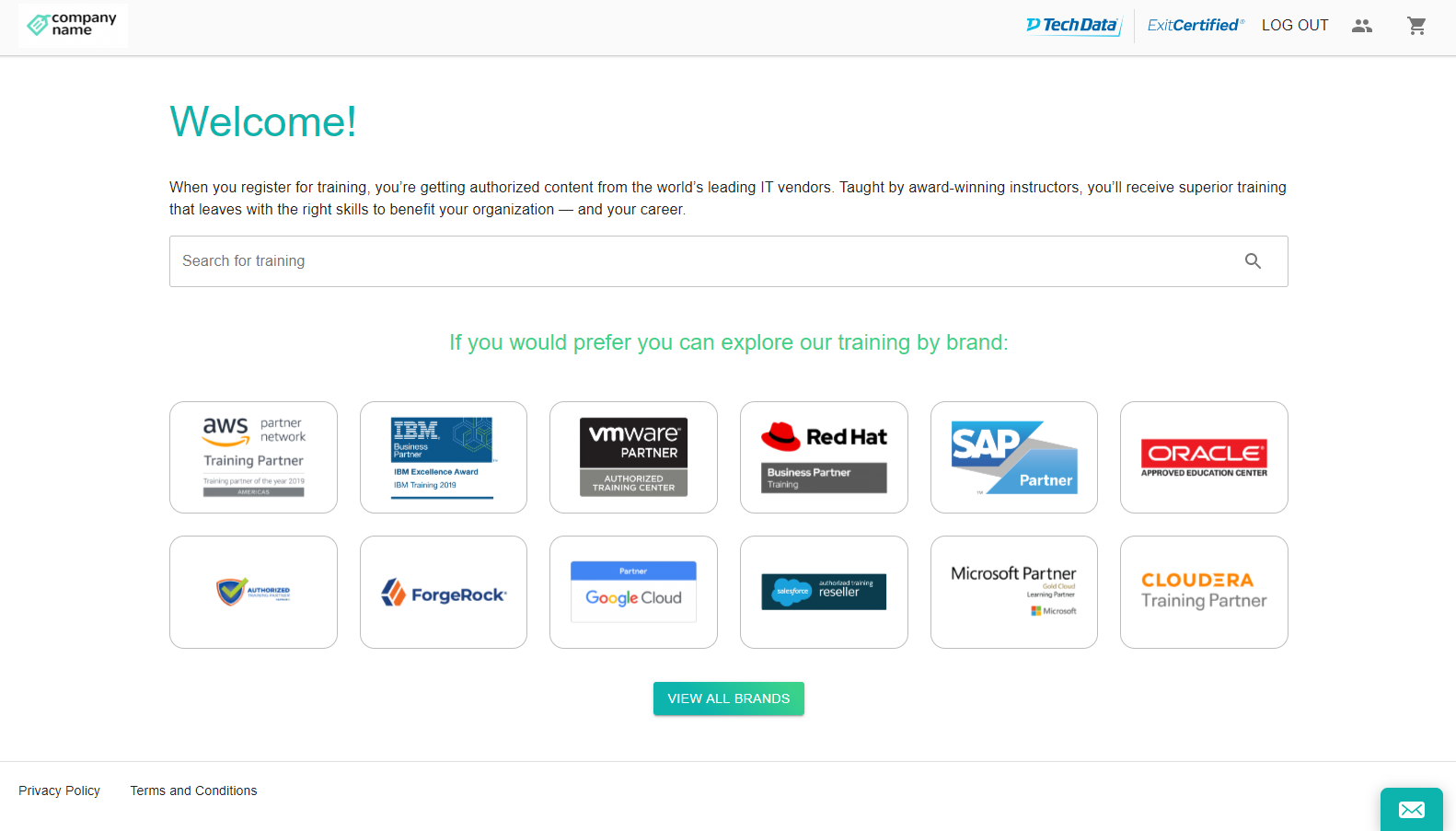This image is a screenshot from a company’s training platform. In the top left corner, it displays the company name. Below this are several navigation options: "Tech Data," "Exit," "Certified," and "Log out." Next to these options are two icons depicting people from the shoulders up, and a shopping cart icon with the label "Welcome."

The main section of the page informs users about the benefits of registering for training on this platform. It states that registrants will receive authorized content from the world's leading IT vendors, taught by award-winning instructors. This training aims to provide superior skills that will benefit both individual careers and organizations.

Below this information, there is a search bar with a magnifying glass icon, along with a message suggesting users can explore training options by brand. The brands listed include:

- AWS (Amazon Web Services), indicated by the Amazon brand training partner logo
- IBM, represented by a blue logo
- VMware, Red Hat, and SAP, all labeled as partners
- Oracle, marked with a red logo
- A logo resembling a tiny blue shield with a green checkmark
- ForgeRock
- Google Cloud, highlighted with a dark blue banner and a light blue cloud
- A partially readable logo suggesting the words "Researcher" or "Reseller"
- Microsoft Partner
- Cloudera Training Partner

Each of these brands is visually represented by distinct logos.